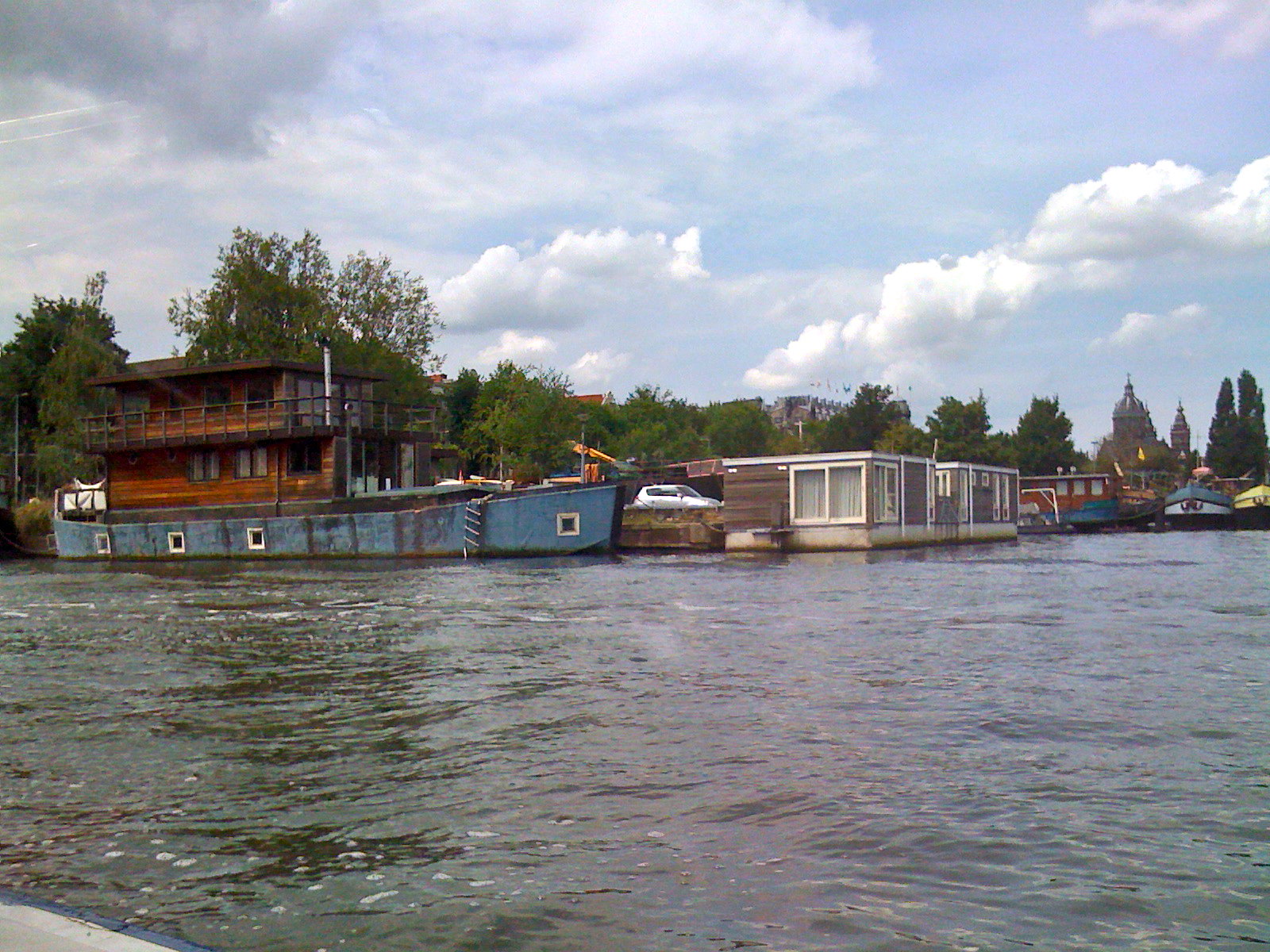The photograph captures a scenic harbor scene featuring calm, rippling water occupying the lower portion of the image. On this tranquil water, there are two prominent houseboats. The larger houseboat to the left has a blue hull and features a wooden, two-story house on top, complete with a wraparound deck on the second level. The houseboat on the right is more square-shaped, with light brown walls and large white windows, suggesting a cozy living space. 

Behind these houseboats, a small blue car is visible on what appears to be a dock or the shore. The shoreline is adorned with green trees and additional small buildings, likely residences either on the water or adjacent to it. In the middle of the image, further in the background, more boats can be seen, adding to the bustling harbor atmosphere.

The upper part of the image showcases signs of human habitation, with more buildings and a grander structure featuring domes and flags, possibly hinting at a European location. The sky above is mostly cloudy, with patches of blue peeking through, creating a picturesque backdrop to the peaceful waterfront setting.